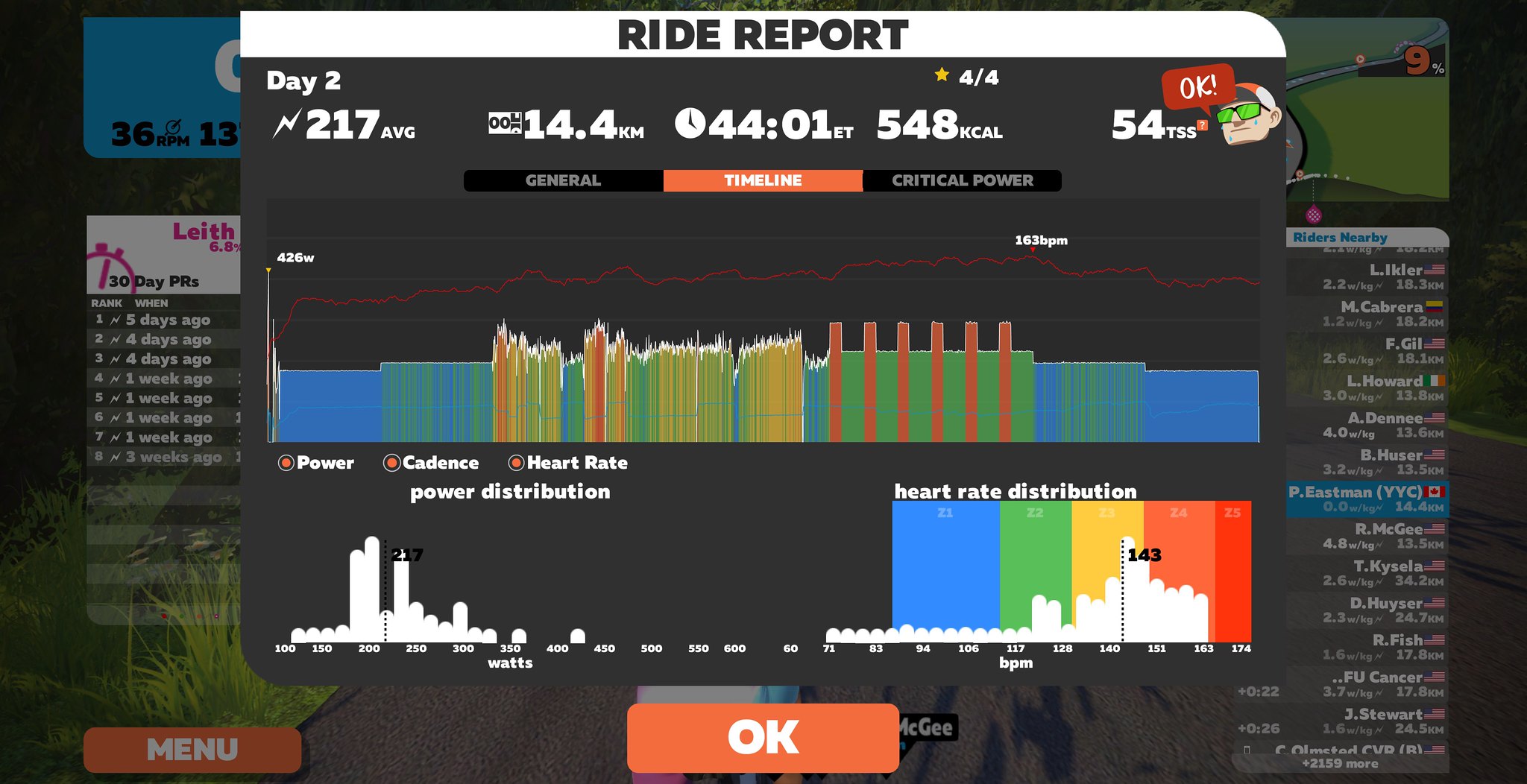This detailed screenshot from a workout app displays comprehensive metrics for a bike riding session. At the top, the white-highlighted header reads "Ride Report," and just below, the green square indicates "Day 2" with an average of 217 watts over a distance of 14.5 kilometers. The clock icon shows the duration as 44:01 (44 minutes and 1 second), with a total calorie burn of 548 kcal. Next to this, a red square denotes "54 TSS," and a cartoon face with green sunglasses and a red and white hat provides a playful element. In the center, a multicolored bar graph (blue, yellow, orange, and red) represents different workout intensities, with a line graph overlay to show performance trends. Below this, a tiny white bar graph tracks another aspect of the workout, likely related to heart rate, which is detailed below the main graph. In the lower left corner, average generated power is indicated as 217 watts. To the lower right, a rainbow-colored graph adds visual diversity. The background features a faded gray board with white text, while a prominent red "Okay" button appears at the bottom to finalize the report.